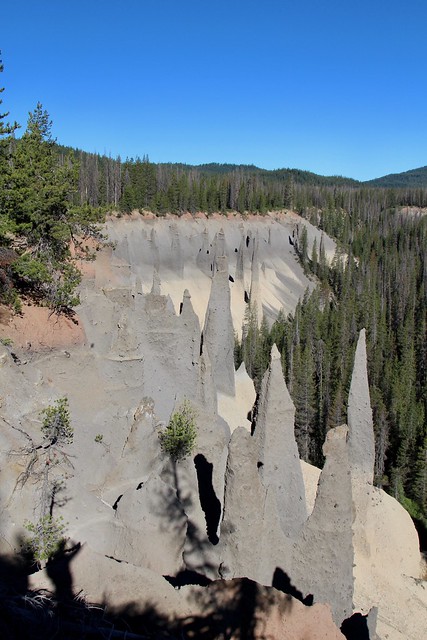The photograph captures a striking natural landscape likely from Yellowstone National Park or a scenic locale in Colorado. Dominating the scene are towering evergreen trees and tall, slender pine trees, their green leaves interspersed with patches of gray and brown vegetation. This dense forest surrounds a canyon filled with large, triangular, or pyramidal rock spires that rise majestically from the ground. These rock formations vary in color from gray to shades of tan, dark red, and clay. The forest floor beneath the trees transitions from pinkish and brown dirt to ash-gray rock. The clear blue sky forms a vivid backdrop, unblemished by clouds. Shadows cast by visitors, including one distinctly showing a person with a backpack, add a subtle human element to the majestic natural setting.